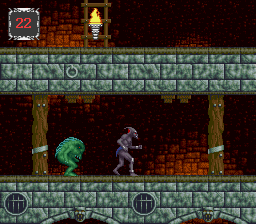This captivating still from a video game depicts a scene set within a multi-leveled dungeon. The dungeon's architecture features a rich red brick background and sturdy gray cobblestone floors, adding a gritty texture to the environment. One of the levels is supported by large, wooden pillars, giving it a robust and medieval feel. The dungeon walls are lined with sconces, each emitting a warm, yellow flame that illuminates the dimly lit space. A wooden ladder provides a means to traverse between the levels. In the top corner of the image, the number "22" is prominently displayed, likely indicating a level or area number. On the bottom level, two intriguing characters are seen walking side by side: a round, green monster and a muscular, purple demon-like creature, adding a sense of adventure and challenge to the scene.